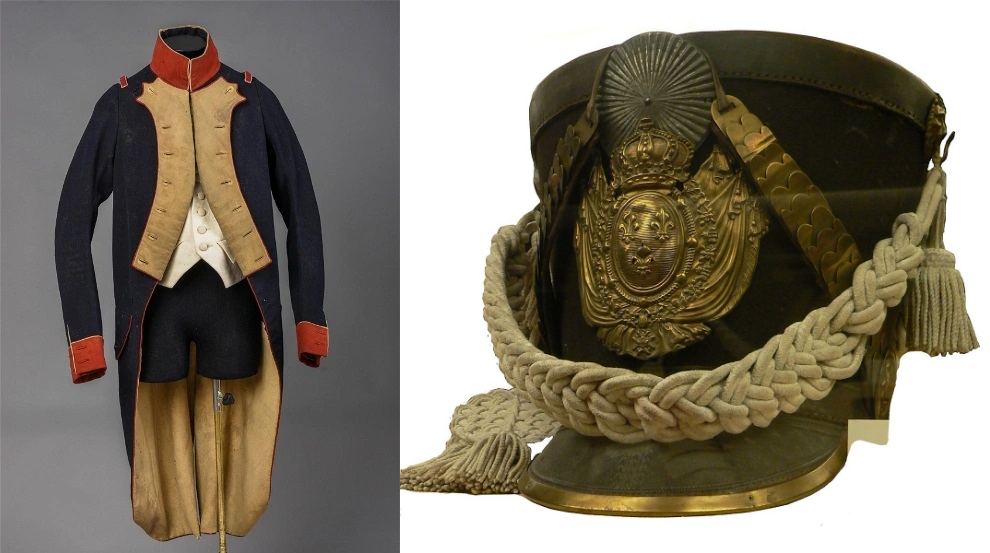The image displays two pieces of a soldier's uniform from the colonial era. On the left side is a distinguished military overcoat, primarily dark blue in color, extending to the hamstrings at the back. The overcoat features maroon accents on the collar and cuffs, as well as a tan central flap adorned with buttons. Underneath, a white vest is partially visible, and below that, the soldier appears to be wearing black shorts. 

On the right side of the image is an ornate helmet, predominantly green with intricate details. A gold crest decorates the front, complemented by a braided white rope that extends around the sides to the front. The visor of the helmet has a gold border, adding to its elaborate design. The helmet, like the coat, exudes a sense of historical military grandeur, indicative of the colonial era.